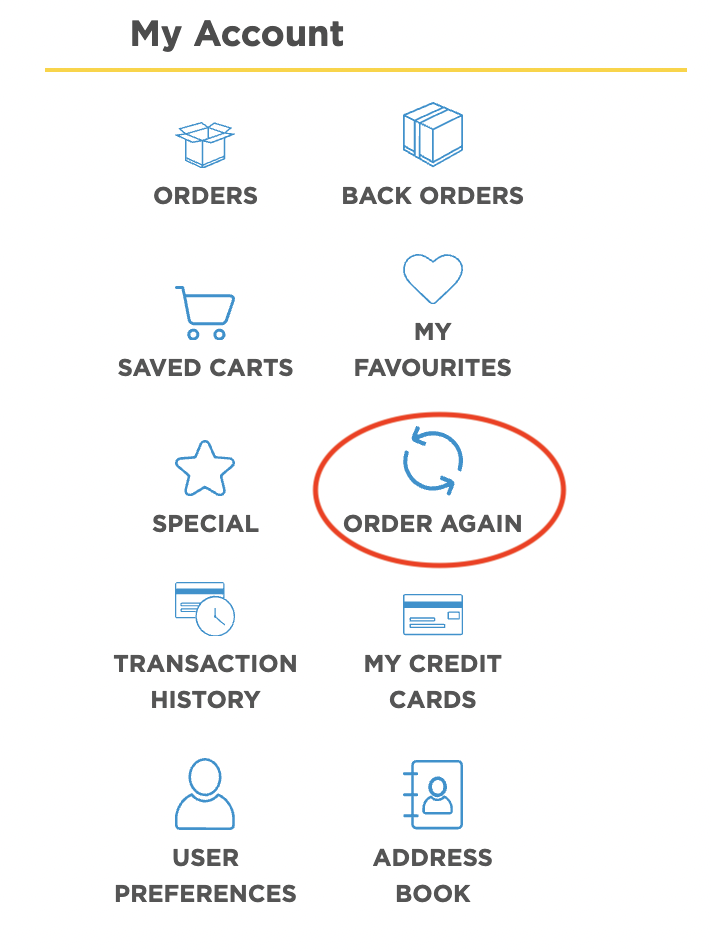At the top of the page, there is a bold black text that reads "My Account," with a distinctive yellow line underneath. Below this header is an image of an open box outlined in blue, accompanied by the word "ORDERS" in all uppercase text.

To the right, there is an image of a closed box with the label "Back Orders" written in black text underneath. Moving downward, there is an icon of a shopping cart with the text "Saved Carts" below it. Next, a heart icon symbolizes "My Favorites," followed by a star icon with the word "Special" underneath it.

Prominently highlighted in red is a circular arrangement featuring two arrows, one pointing left and the other right. This circled area focuses attention on the option "Order Again." Below this, "Transaction History" is indicated by an image of a credit card with a clock in front of it. 

Further down, there's an icon of a blue credit card labeled "My Credit Cards." An image depicting the silhouette of a person's face and upper body represents "User Preferences." Finally, the "Address Book" is visualized by an icon resembling a book with a silhouette of a person's face on its cover.